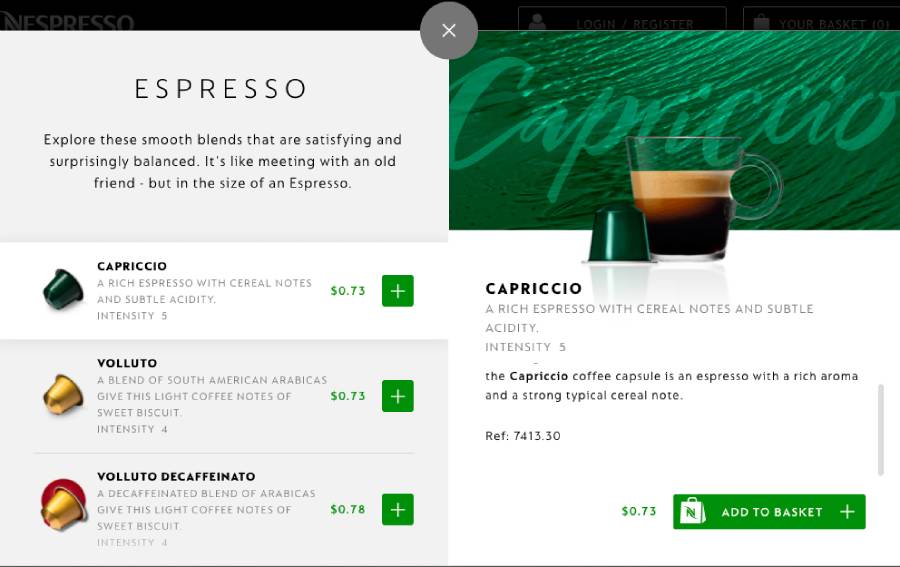The rectangular image captures a detailed view of a coffee-related website, either a marketplace for coffee products or an online restaurant menu. 

On the left side of the website, a pop-up window prominently displays the bold, all-capital word "ESPRESSO" in black text. Below this heading, there is a short, enticing description that reads: "Explore these smooth blends that are satisfying and surprisingly balanced. It's like meeting with an old friend, but in the size of an espresso." 

Beneath this introductory text, a list of various espresso varieties is presented, with each name bolded in black font and accompanied by individual descriptions. Adjacent to the list, images of the corresponding espresso pods, which resemble K-Cups for instant coffee makers, are displayed. The first pod is dark green, followed by two gold-colored pods.

The right side of the website showcases the main content area. The upper third features a dark green background with the word "Capriccio" written in a cursive, lighter green font. Below this, a clear glass mug displays a layered espresso drink, with a light brown layer atop a dark brown layer, sitting next to an upside-down dark green K-Cup.

Further down, a thin, rectangular green button with white text is visible. To the left of the button, an icon of a shopping bag is displayed. The button itself is labeled "Add to Basket" in white, with a small plus sign to the right.